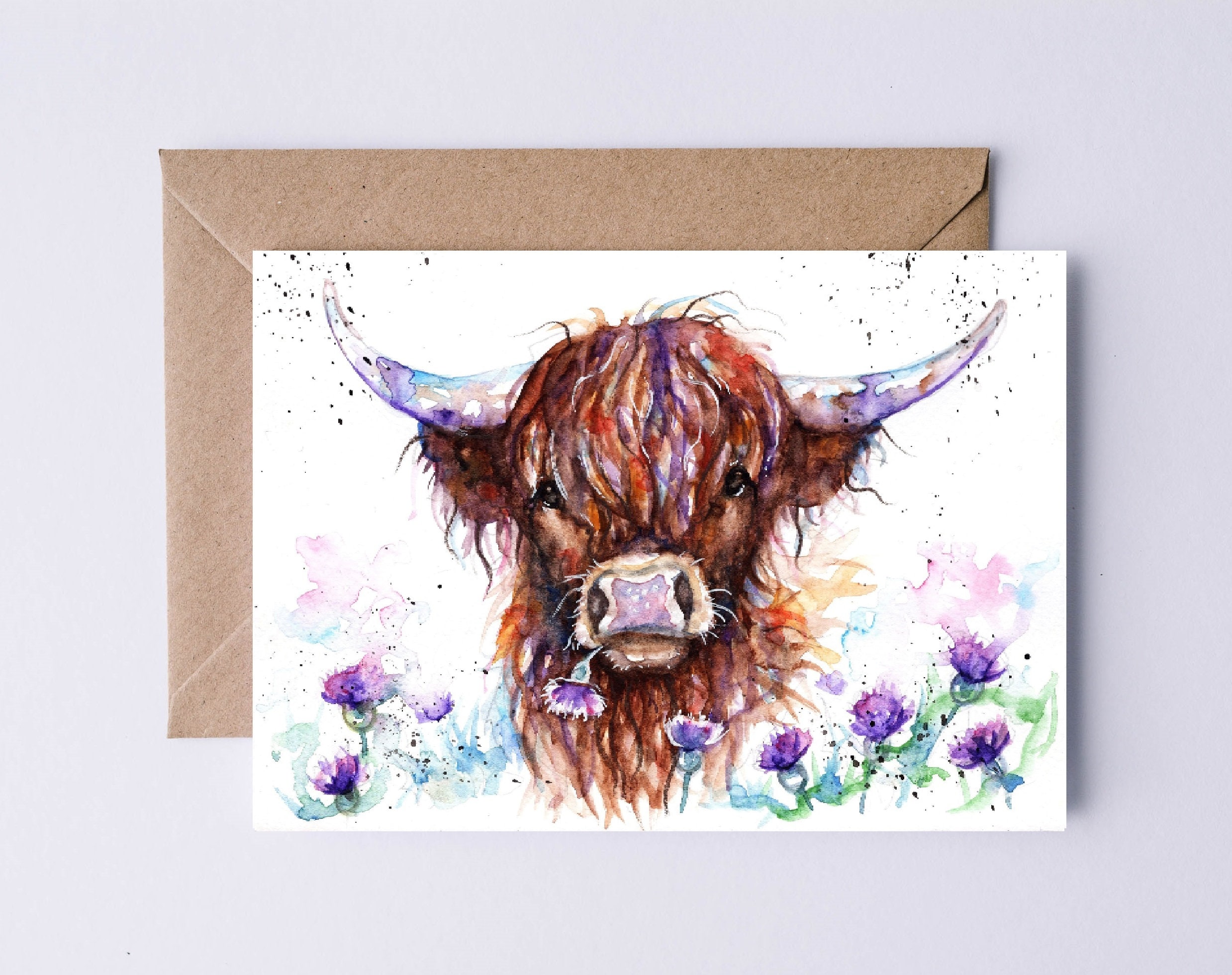The image showcases a hand-painted watercolor greeting card featuring a young Highlands bull with long, white horns and brown fur streaked with purple. The bull, with expressive brown eyes and a large cream-colored nose, is depicted chewing on a blue flower that hangs from its mouth while looking directly at the observer. Surrounding the bull are several upright blue flowers, adding a botanical touch. The white background of the card is subtly splotched with hues of pink, yellow, green, and blue from the watercolor. The card is positioned on a light lavender surface, with a brown paper envelope placed behind it, matching its size and adding a rustic feel to the scene.